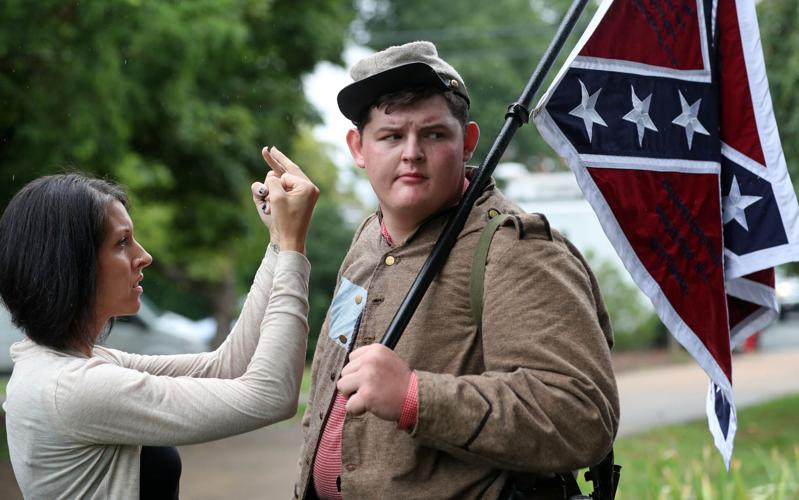The photograph captures a stark moment of political tension and emotional confrontation. In the image, a middle-aged woman with short, medium-length dark hair, dressed in a relatively thin white cardigan or sweater over a black shirt, stands on the left. She holds both her middle fingers up inches away from the face of a young, pudgy white man, who appears to be in his late teens or early 20s. The man, who seems overweight, is wearing a brown button-up sweater with a red polo, or possibly a red and white striped shirt underneath. His sweater is buttoned at the top with the rest hanging open. He also has a gray, somewhat lopsided newsboy cap on his head and carries a large Confederate flag over his shoulder, trailing behind him. Despite the woman's visibly furious gesture directed right at him, the man pointedly looks away to the right, frowning and appearing disinterested. He is also equipped with a green satchel or backpack. The backdrop of the scene is a sunny outdoor setting with abundant greenery. The contrasting expressions and body language of the two individuals highlight the intense disagreement and charged atmosphere captured in this photograph.